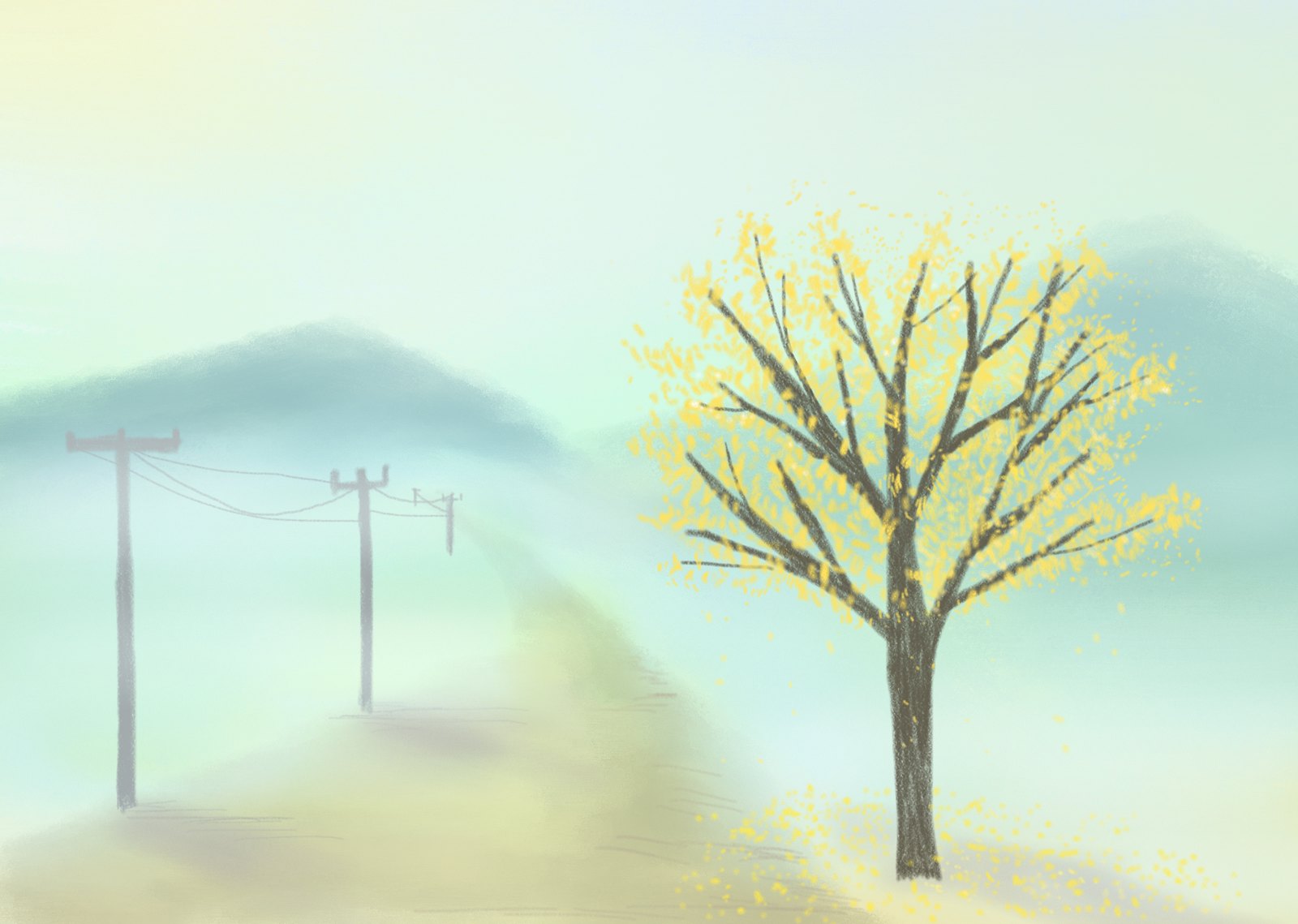A captivating digital artwork exuding a fantastical, ethereal quality. To the right, a tree with twisting brown branches adorned with yellow leaves that flutter to the ground. On the left, a gravel road stretches into the distance, bordered by a series of power lines. Mountains painted in a unique greenish-blue palette rise majestically in the background, blending harmoniously with the yellow-tinged sky. The entire scene is enveloped in a soft, foggy atmosphere, enhancing its otherworldly charm.